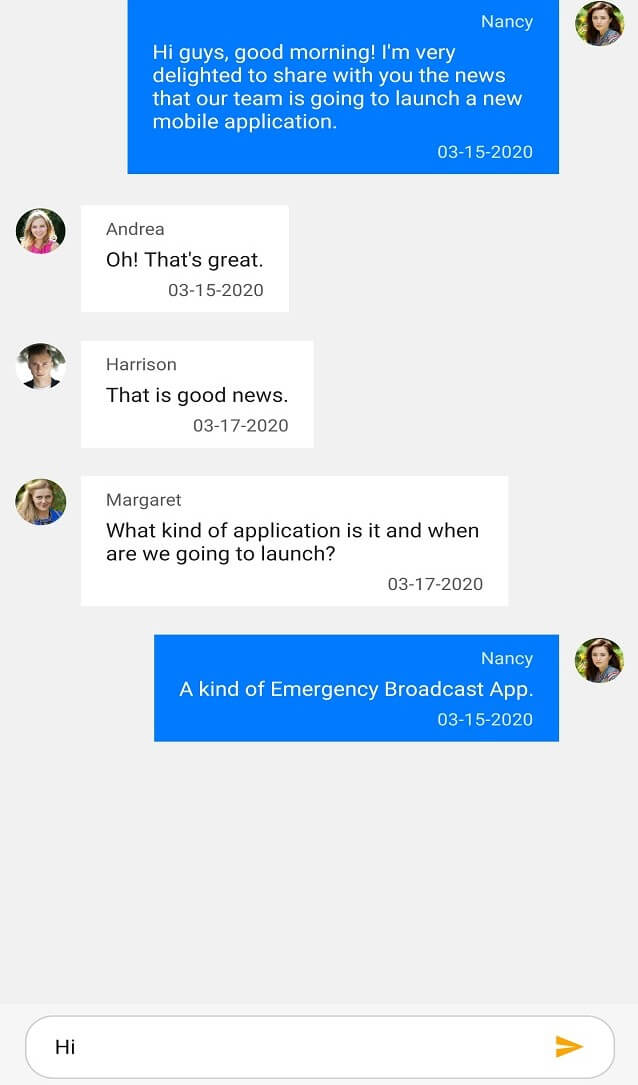The screenshot displays a group chat conversation on a gray background. Here's a detailed breakdown:

- **Top Right Corner:**
  - **User:** Nancy
  - **Background:** Blue
  - **Text:** White
  - **Message:** "Hi guys, good morning. I'm very delighted to share with you the news that our team is going to launch a new mobile application."
  - **Timestamp:** 03/15/2020

- **Below Nancy's Message:**
  - **User:** Nancy
  - **Picture:** A white female with dark brown hair, looking directly at the camera.
  
- **Next Message:** 
  - **User:** Andrea (A blonde with a pink shirt)
  - **Message:** "Oh, that's great."
  - **Timestamp:** Same day, in gray text.

- **Next Message:**
  - **User:** Harrison (A white male with a slight smirk looking straight ahead)
  - **Message:** "That's great news."

- **Further Conversation:**
  - **User:** Margaret (Another blonde)
  - **Message:** "What kind of application is it and when are we going to launch?"
  
- **Nancy's Reply:**
  - **Message:** "A kind of emergency broadcast app. Do you need an emergency broadcast app for...?"

- **Final Element of the Screenshot:**
  - **Reply Box:** Features a black "Hi" with a blue and yellow 'Send' button on the right-hand side.

The image effectively captures a conversation about the launch of a new mobile application, demonstrating the excitement and curiosity of the involved team members.